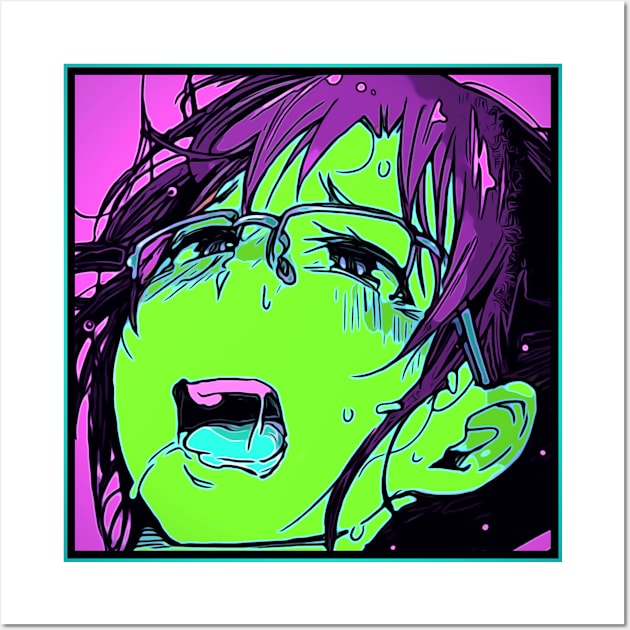This detailed digital artwork features an anime-style young girl with striking purple hair adorned with small polka dots. She has short, messy bangs, and her hair length reaches down to her chin. The girl's face is an unusual bright lime green, complemented by her purple lips and blue tongue. Her eyes, encased in light-rimmed glasses that cover only the top and sides, express a mix of intense distress and pleasure, evidenced by the tears streaming down her face and the sweat dripping from her forehead. Her mouth is open wide, showcasing her pink teeth, with drool cascading from the corners down to her chin. Positioned as if lying on her back and looking upward, she is set against a pink background, contributing to the image's vivid emotional intensity.